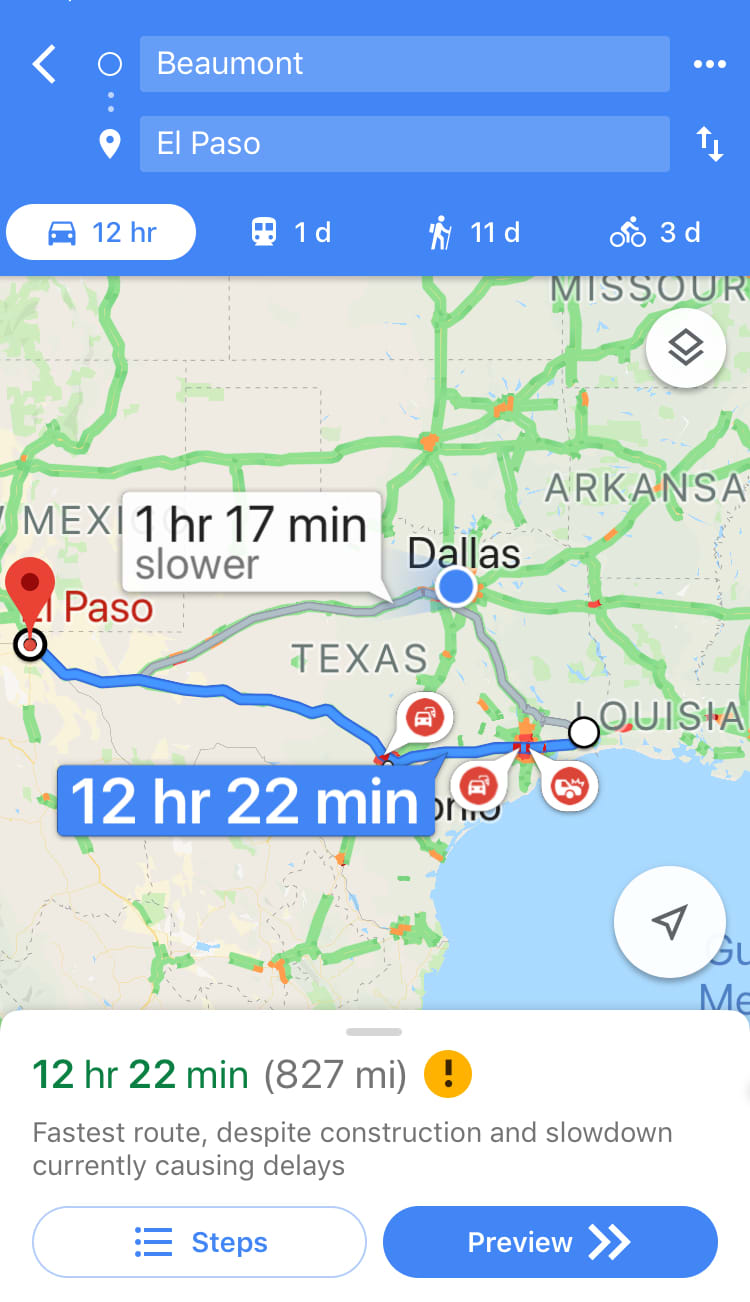A screenshot from the Google Maps app displays a detailed route plan from Beaumont to El Paso. At the top is a light blue navigation bar that includes a left-pointing arrow for returning to the previous screen, a search bar, and a menu icon composed of three horizontal dots. Directly beneath, still within the blue box, are various transportation icons with corresponding travel times: a car (12 hours), a train (one day), a pedestrian (11 days), and a cyclist (three days). The car option is selected, indicating a 12-hour drive.

Below the navigation bar, the map illustrates two highlighted routes from Beaumont to El Paso. The primary route is marked at 12 hours and 22 minutes, while an alternative route is indicated to be one hour and 17 minutes slower. At the bottom of the map, more detailed information states, "12 hours, 22 minutes, 827 miles!" It highlights that this is the fastest route despite construction and delays.

Finally, the interface includes two oval buttons at the bottom: a white one with blue text labeled "Steps" accompanied by a menu icon, and a blue one with white text labeled "Preview," featuring two forward-pointing arrows.